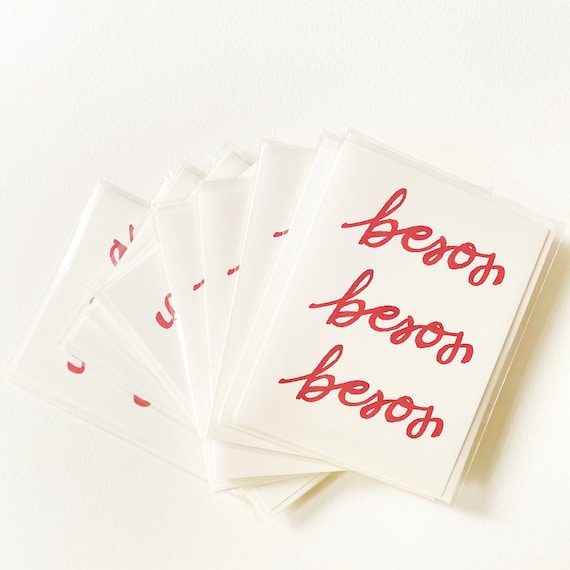The image depicts a stack of white greeting cards fanned out against a white background, creating a subtle shadow effect that highlights the edges of the cards. At the top of the stack is an exposed card displaying the word "Besos" written in red cursive script, repeated three times down the length of the card. While you cannot see the details of the cards underneath, it is implied that they share the same design. The stack also contains white envelopes nestled between the cards, contributing to the overall orderly but slightly staggered arrangement. The repetition of the cursive "Besos" and the crisp white aesthetic emphasize a cohesive and elegant theme throughout the image.